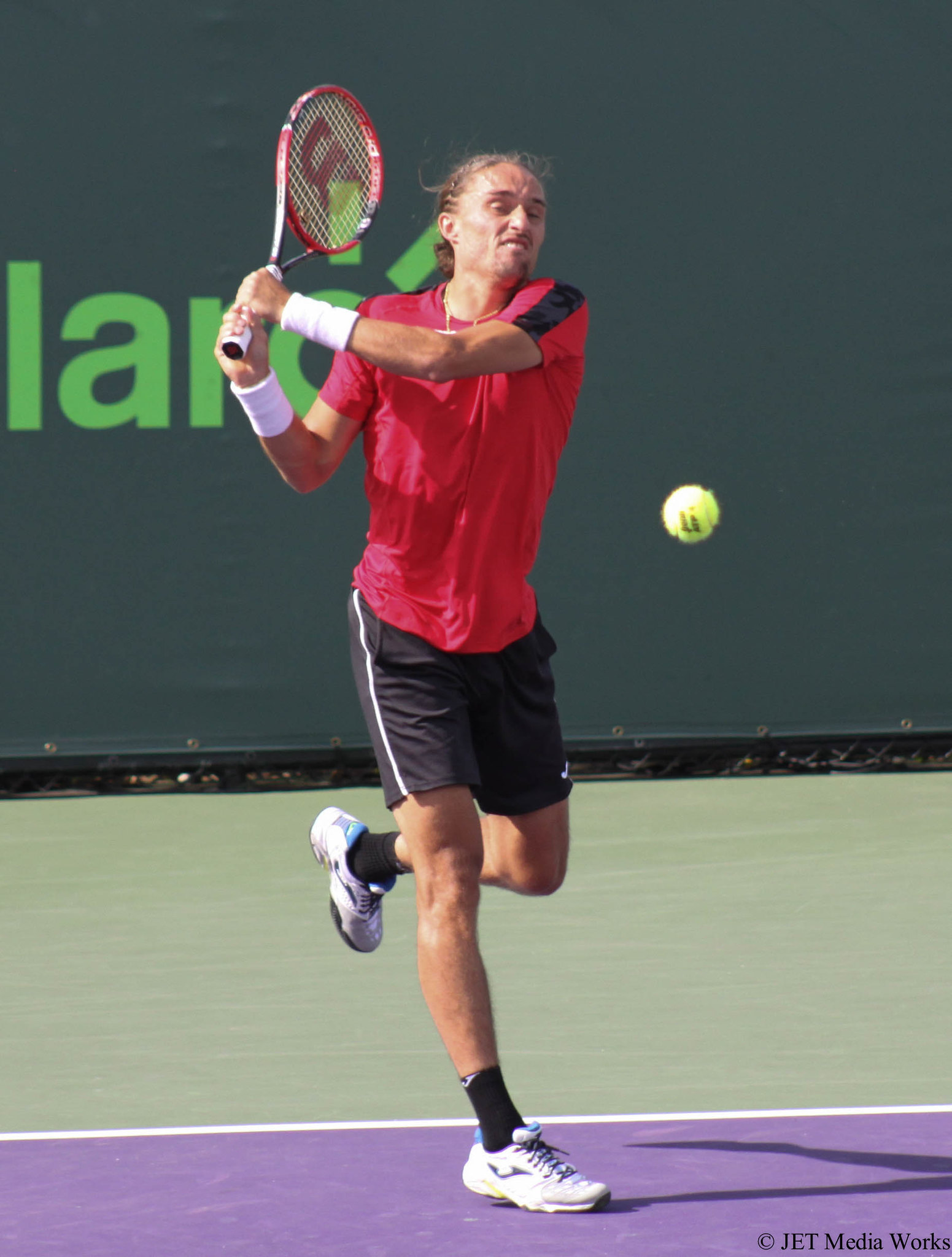In this vibrant outdoor color photograph, a tennis player with long brown hair tied in a ponytail is captured mid-action, having just hit the ball, which hovers in the air to the right. Demonstrating intense effort with a grimace, he stands on one leg while the other trails behind. His racket is poised over his left shoulder, held with both hands. He sports a red shirt with black stripes, black shorts featuring thin white stripes, white wristbands, black socks, and white sneakers. The player is positioned on a distinctive purple tennis court, bordered by a light green section, with a dark gray or black wall in the distant background. This wall is adorned with large, light green letters, likely spelling "L-A-R-C," and labeled in small black text with "Jet Media Works" in the lower right corner.